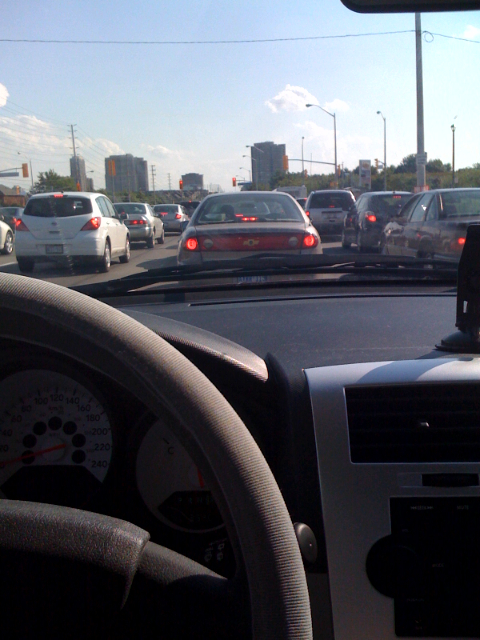This photograph, taken from inside a car during rush hour traffic, captures the palpable congestion of the moment. The vantage point is from the driver's seat, with the steering wheel positioned on the left side, adorned with a sleek black fabric-covered steering wheel cover. The interior of the car is predominantly black, giving it a modern yet subdued aesthetic, with a touch of silver detailing around the radio area on the dashboard.

Central to the dashboard is a mount, likely for a GPS device or a cell phone, strategically placed above the media console to aid in navigation. The scene outside the windshield reveals the heavy traffic, with cars lined up in at least four lanes, each vehicle's crimson brake lights glowing in unison, signaling the halt imposed by the red stoplight visible in the distance.

Adding to the urban landscape, four tall, older-style apartment buildings rise in the background, standing as silent witnesses to the daily ebb and flow of city life. The buildings' worn facades contrast against the modern congestion of vehicles, highlighting the city's blend of historical architecture and contemporary challenges.